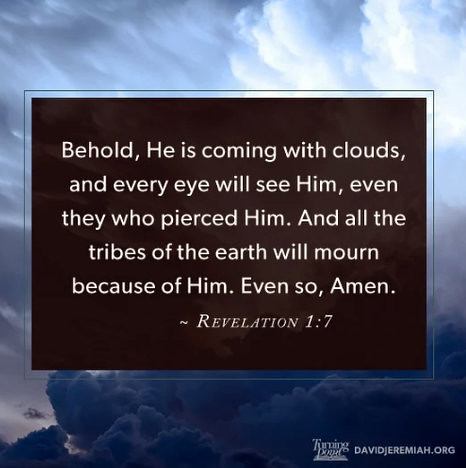The image is a square photograph of a cloudy sky, featuring a gradient from dark clouds at the bottom to lighter clouds at the top. Superimposed over this background is a smaller square with a narrow, one-pixel-wide black border. The square itself has a solid black background and contains medium-sized white text in the center, which reads: “Behold, he is coming with clouds, and every eye will see him, even they who pierced him. And all the tribes of the earth will mourn because of him. Even so, Amen. Revelation 1:7.” At the bottom right corner of the photo, small text reads “DavidJeremiah.org” alongside a logo for Turning Point. The overall design gives off a religious and reflective tone, commonly seen in inspirational social media graphics.